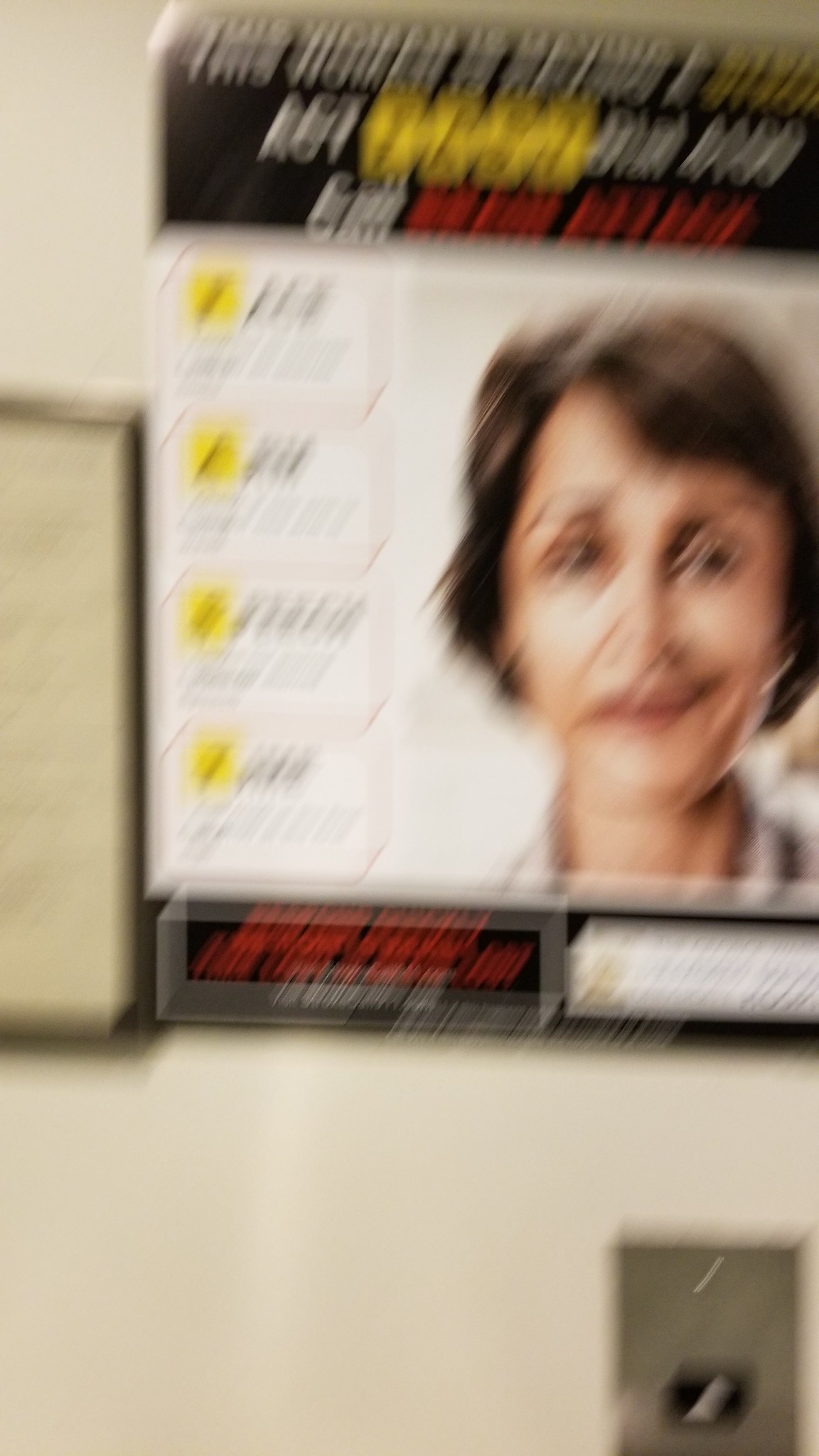This is a blurry color photograph of an indoor setting, primarily featuring a white wall and a door. Dominating the scene is a door equipped with a silver handle positioned near the bottom right corner. Adjacent to the handle is a silver rectangular object, potentially a wall plate or light switch. A poster is mounted on the door, exhibiting an image of a woman believed to be a doctor, identifiable by her white coat and stethoscope. The woman, who has short brown hair and brown eyes, appears to have accompanying text that is too indistinct to decipher. The upper section of the poster states, “This woman is something,” though the remainder is illegible. In the poster's right section, the doctor’s image is seen, and on the left, there are four boxed sections bordered in red. Each section contains yellow squares at the top left, followed by black text. Below these, several areas include illegible text in different colors—white, red, and yellow—over varying backgrounds. Additionally, there is a small picture frame on the door with a silver frame and a white, blank interior. The overall composition, though the details remain fuzzy, suggests informational content, possibly outlining procedures, services, or a step-by-step guide.